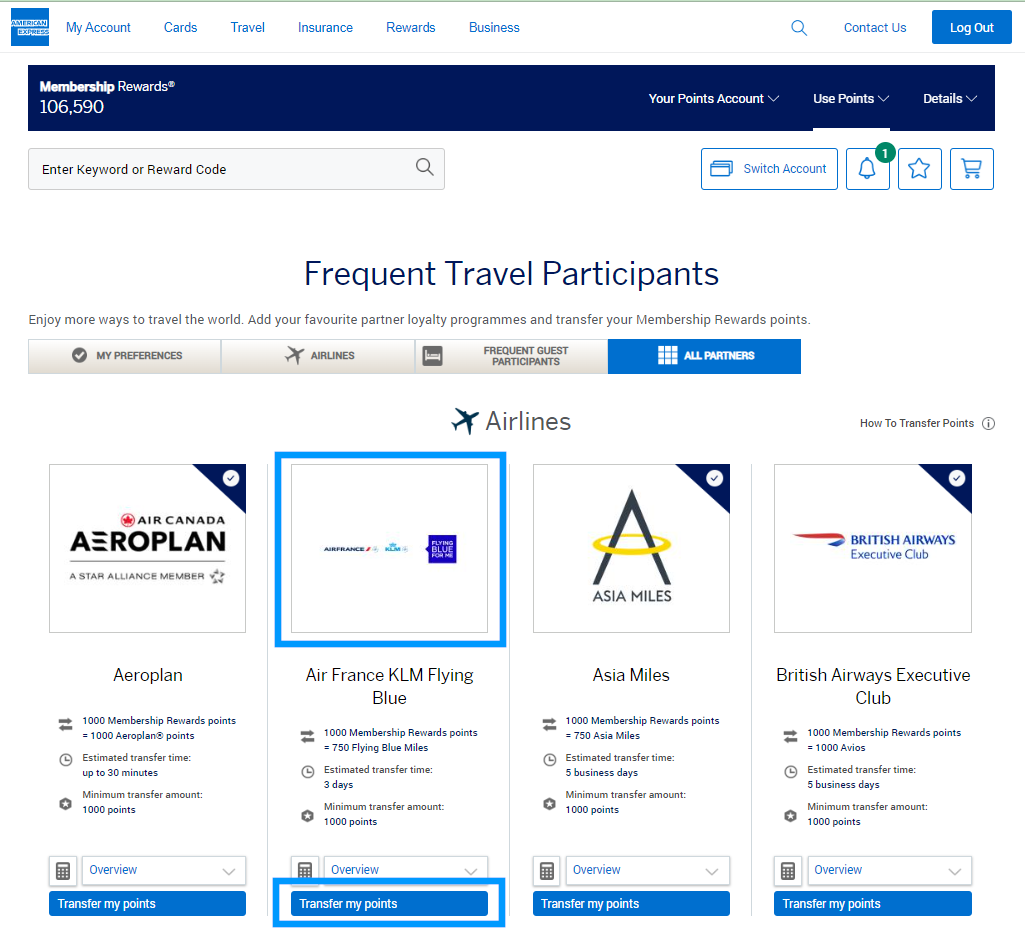This image showcases a web page from American Express. In the upper left-hand corner, the iconic American Express logo is displayed, consisting of a blue square with the words "American Express" in white text, framed by a white border. The rest of the screen has a clean, white background. 

At the top of the screen, a navigation bar spans from left to right, featuring menu options such as "My Account," "Cards," "Travel," "Insurance," "Rewards," and "Business." On the far right, you'll find a magnifying glass search icon, a "Contact Us" link, and a prominent blue button labeled "Log Out" in white text.

Beneath this navigation bar, a navy blue ribbon stretches across the page. On the far left of this ribbon, in white text, it displays "Membership Rewards" along with "106,590" points. On the far right, it reads "Your Points Account" with links to "User Points" and "Details," all in white text.

Further down, the main content section continues with a white background. On the far left, there is a light gray search bar with placeholder text in gray that says "Enter keyword or reward code." To the right of the search bar are various options presented as white buttons outlined in bright blue, including "Switch Account," a notification bell showing one alert, a star, and a shopping cart icon.

In the center of the page, prominently displayed in navy blue text, is the heading "Frequent Travel Participants." Below this, in light gray text, it reads "Enjoy more ways to travel the world, add your favorite partner loyalty programs, and transfer your Membership Rewards points." 

Under this introduction, there are four boxes: one labeled "My Preferences," followed by "Airlines," "Frequent Guest Participants," and a bright blue button with white text that reads "All Partners." The first three boxes are light gray with dark gray text.

Lastly, towards the bottom of the page, "Airlines" is centered with a plane icon next to the word. Four featured airlines are displayed: Air Canada Aeroplan, Air France KLM Flying Blue, Asia Miles, and British Airways Executive Club.